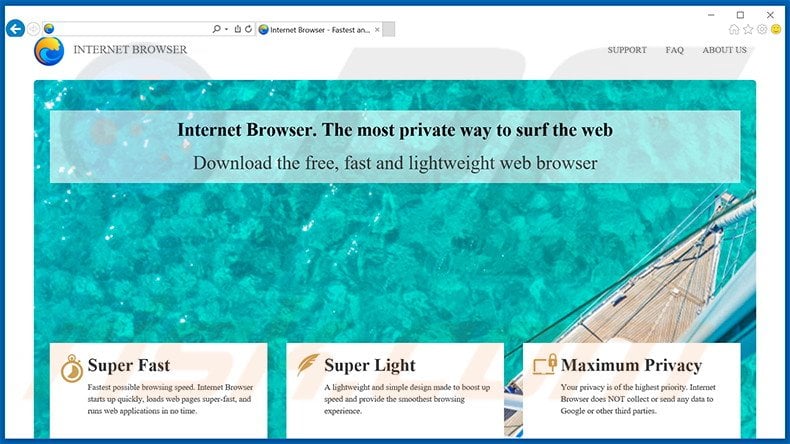The screenshot captures an internet browser interface. In the upper left-hand corner, there is a back button followed by a URL bar, with a single open tab displaying a website titled "Internet Browser." On the upper right-hand side are the close (X), minimize, and reduce size buttons.

Below these controls, a row of icons is visible: an emoji icon, a gear icon, a star icon, and a home icon. The website loaded in the browser prominently displays "Internet Browser" in the upper left along with a wave icon emblematic of the browser. In the upper right, there are three navigational buttons labeled "Support," "FAQ," and "About Us." 

The website's background image features a top-down view of a sailing ship navigating a vividly blue ocean. Superimposed on this backdrop is a text that reads, "Internet Browser: The most private way to surf the web." Additional text promotes the browser as a free, fast, and lightweight option for browsing.

Towards the bottom of the webpage, three white text boxes provide further details:
1. The first box, titled "Super Fast," highlights the browser's quick startup, rapid page loading, and efficient web application performance.
2. The second box, "Super Light," emphasizes the browser's lightweight and simple design, engineered to enhance speed and ensure a seamless browsing experience.
3. The third box, "Maximum Privacy," assures users that their privacy is a top priority, stating that "Internet Browser" does not collect or transmit any data to Google or other third parties.